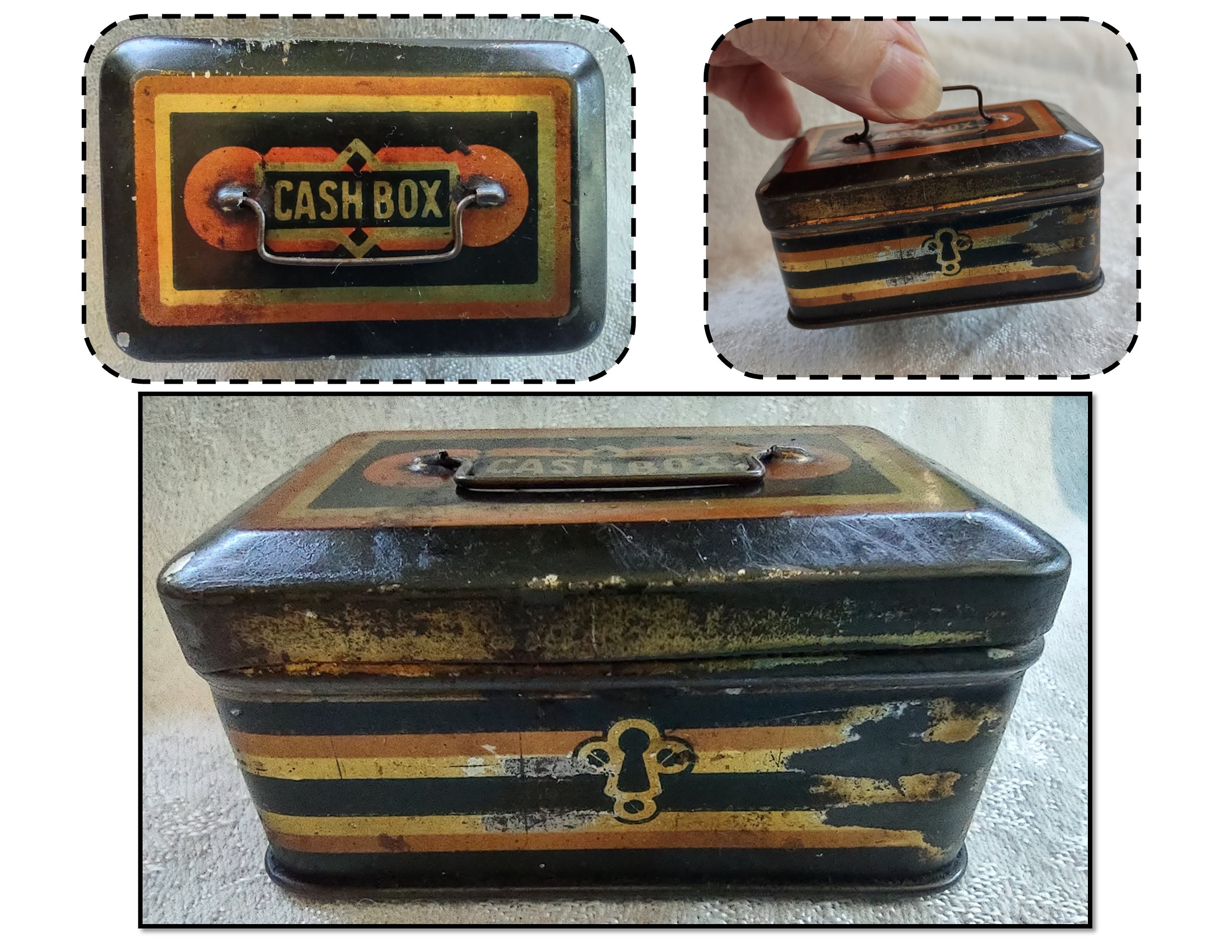The image is a collage of three photographs, each depicting different views of a small, aged metal cash box. The bottom photograph is the largest and shows a close-up frontal view of the cash box, which is framed by a solid black border. The box is old, rough, and rusted, with a beat-up appearance. It features a faux keyhole illustration in black, orange, and yellow, and the words "cash box" are prominently displayed on the top. The two upper photographs are surrounded by dotted black lines. The top left image offers an overhead view of the box, highlighting its worn surface, silver handle, and colorful design consisting of black, orange, and yellow stripes. The top right image shows a hand holding the box by its handle, illustrating the box's small size as it fits snugly between the thumb and forefinger, suggesting it could easily be held in the palm of a hand. The overall clarity of the images is high, with bright and well-lit settings.